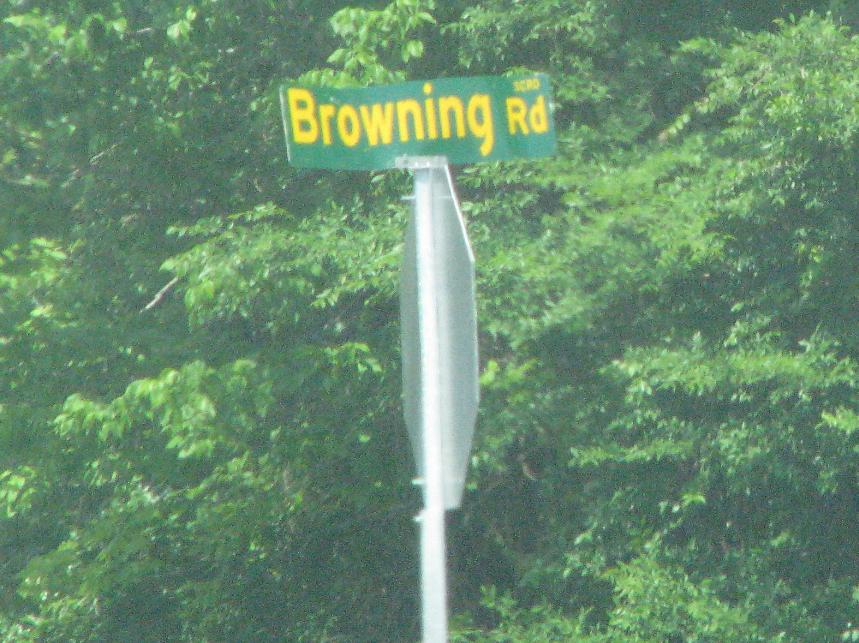This photograph captures a street sign mounted on a stop sign post. The stop sign itself is turned away from the camera, revealing only its gray metallic backing and the characteristic octagonal shape, affixed to a tall, silver cylindrical pole. At the top of this pole, a dark green street sign with bright yellow letters, clearly reads "Browning RD," facing directly towards the viewer. The backdrop is dominated by lush green foliage and tangled branches, suggesting a tree-lined street environment. The overall quality of the image is grainy, obscuring finer details.